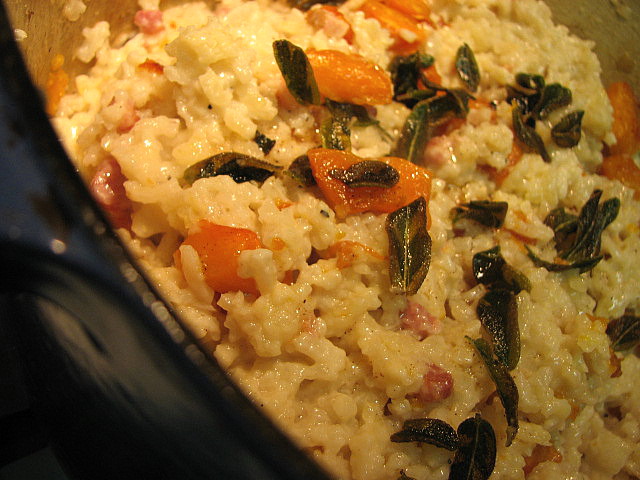The image displays a close-up view of a creamy, thick rice dish, likely risotto, contained in a dark, possibly black or blue bowl with a brown lining visible. The risotto has an opaque, mushy consistency, resembling a thick oatmeal. Scattered throughout the dish are orange chunks, potentially carrots or orange bell peppers, as well as pops of red that could signify either tomatoes or red bell peppers. The dish is garnished with green leaves, which might be fried sage, adding both color and texture to the presentation. The side of the bowl, found at the bottom left-hand corner, reflects light, underscoring the bowl's dark hue.